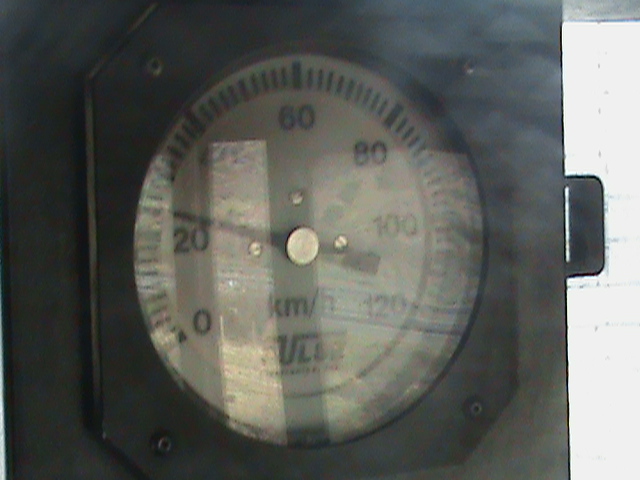This color landscape photograph captures a close-up of a speedometer, which is round with a white face and a prominent black dial. Instead of the traditional 1 through 12 indicating hours, the dial displays speeds from 0 to 120 kilometers per hour. The speedometer currently points to approximately 22 kilometers per hour. Black text encircles the edge of the dial, marking the speed increments. At the bottom of the gauge, there is a indiscernible brand or logo. The glass cover of the speedometer is highly reflective, mirroring an interior scene: the inside of a house with a view of an outdoor setting through three windows. The speedometer's white circular face is enclosed within a black border, which enhances its contrast and highlights the details of the instrument against the darker surroundings.